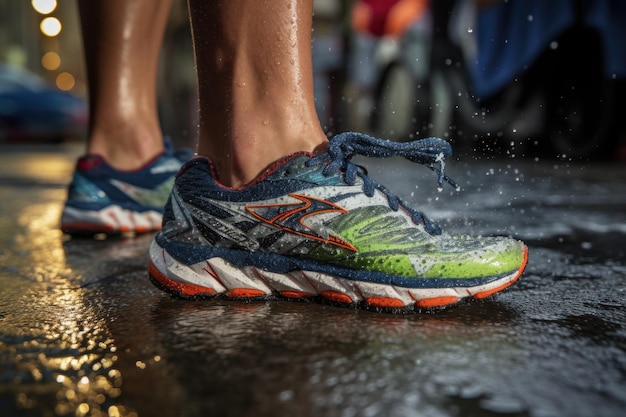This image captures a close-up of a pair of sneakers caught mid-stride on wet pavement, with the environment suggesting a rainy urban setting. The shoes feature thick, multicolored soles—a bright orange bottom layer beneath a white section—and a sophisticated fabric design. The main body of the sneakers includes dark blue fabric with lime green near the toes and an off-white section towards the back, which is adorned with a slate blue-gray swoosh outlined in orange. Dark blue laces complete the footwear's intricate color scheme. Droplets of water are visibly spraying off the person's foot, indicating motion, likely from running. The person's ankles and the shoes appear soaked, further emphasizing that it’s raining. The dark pavement glistens with moisture, and while the background is blurry, you can discern streetlights and a few indistinct objects, adding to the urban atmosphere.